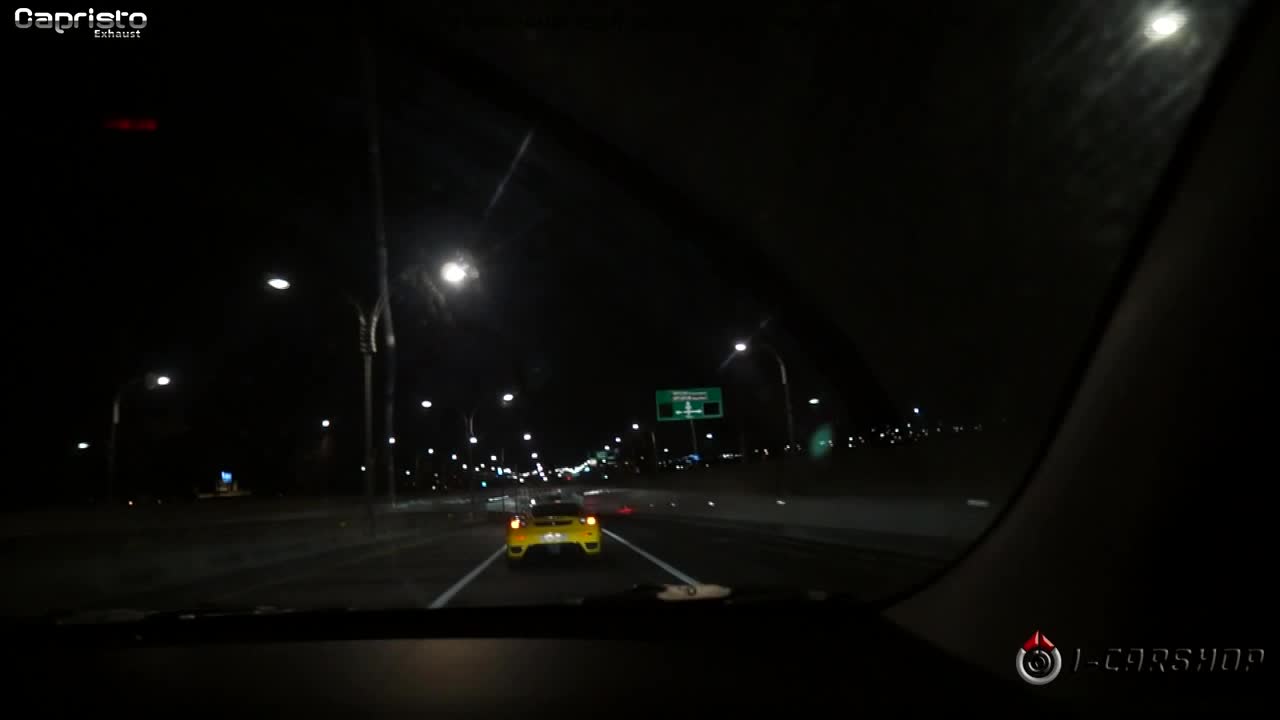A nighttime driving scene captured from inside a car. The sky is pitch black, with numerous streetlights stretching into the distance. In front of the car is a yellow vehicle with illuminated, yellow rear lights. To the right, green street signs indicate lanes, adding realism to the scene reminiscent of a high-tech driving video game. The desolate surroundings are sparsely dotted with buildings and telephone poles. In the top left corner is the word "Capristo," with another smaller, unreadable word beneath it. The right side features an emblem and text, potentially saying "1-car show" or "car shop," along with a gray and red speedometer icon.